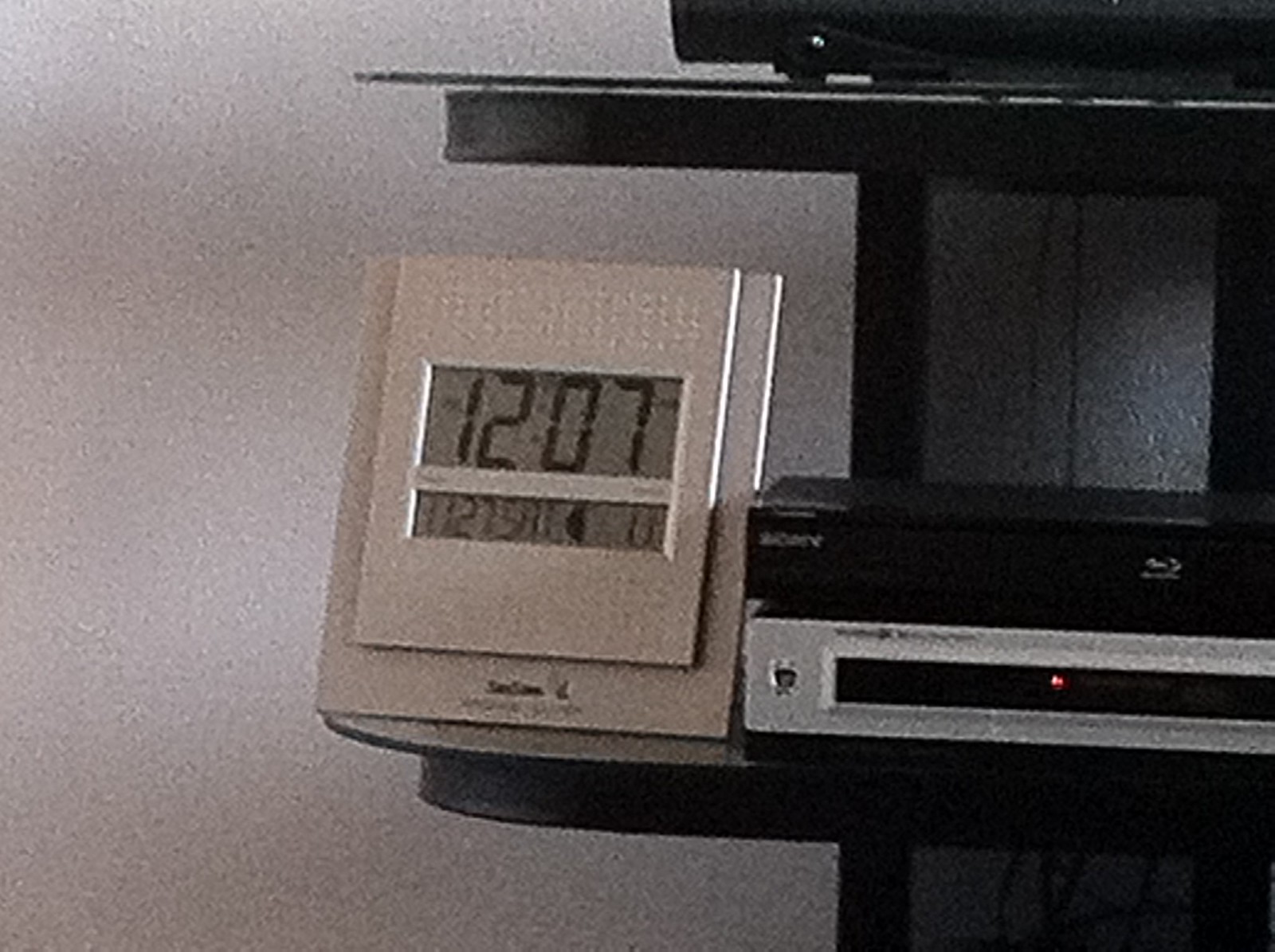The photograph depicts an out-of-focus and slightly grainy image of an entertainment setup, likely in a sitting room. On the left side of the black-colored two-level shelf, there is a large square silver digital clock displaying the time 12:07. Beneath the time, there is an additional, unclear digital display that may show the date and year. Adjacent to the clock on the right is a silver DVD player with a black device—possibly another piece of electronic equipment such as an Xbox or PlayStation—placed on top of it. At the bottom right of the image, part of the shelving unit's legs and a grayish-white wall background are visible. Above the main shelf, part of an upper black shelf is seen with the base of another electronic device atop it. Additionally, several black cords hang down behind the entertainment setup.